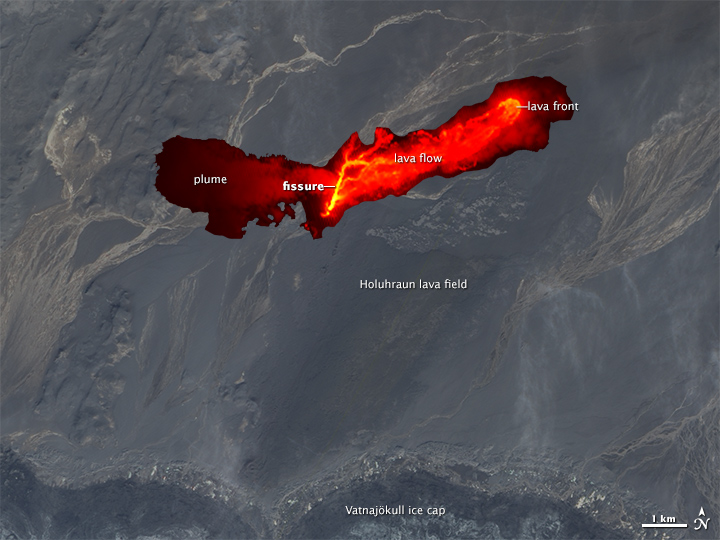The image is an aerial view of a large, predominantly gray, mountainous landscape. Various white labels are overlaid on the image, indicating key features. At the bottom right corner, a white 'N' with an arrow above it points upward, denoting north. To its left, a solid white line is labeled '1 KM' above it, signifying a scale bar. Centered at the bottom of the image, white text denotes 'Vatnajökull Ice Cap.' The central part of the image features stark white text reading 'Holuhraun Lava Field,' referring to a notable volcanic region, characterized by a grayscale mountainous terrain and signs of volcanic activity. A striking bright orange and dark burnt red area at the center marks the site of the eruption and subsequent lava spread, with labels such as 'fissure' pointing towards a yellow lightning bolt-like streak, and 'lava flow' marking the spread of molten rock. Additionally, the word 'plume' is associated with the red portion indicating volcanic emissions.